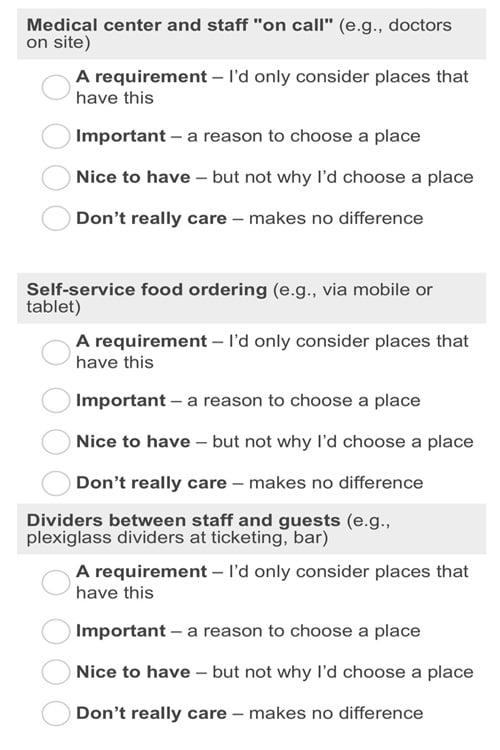The image displays a decision-making survey set against a white background. At the top, there is a light gray banner featuring the dark gray text "Medical center and staff on call," with "doctors on site" emphasized. Below this header, there are four selectable options:

1. "A requirement: I'd only consider places that have this."
2. "Important: A reason to choose a place."
3. "Nice to have: But not why I'd choose a place."
4. "Don't really care: Makes no difference."

Further down, another light gray banner appears with bold black text stating "Self-service food ordering, e.g., via mobile or tablet." This section also offers four selectable answers:

1. "A requirement: I'd only consider places that have this."
2. "Important: A reason to choose a place."
3. "Nice to have: But not why I'd choose a place."
4. "Don't really care: Makes no difference."

The layout is clean and organized, facilitating easy comparison of preferences regarding medical staff availability and self-service food ordering options.